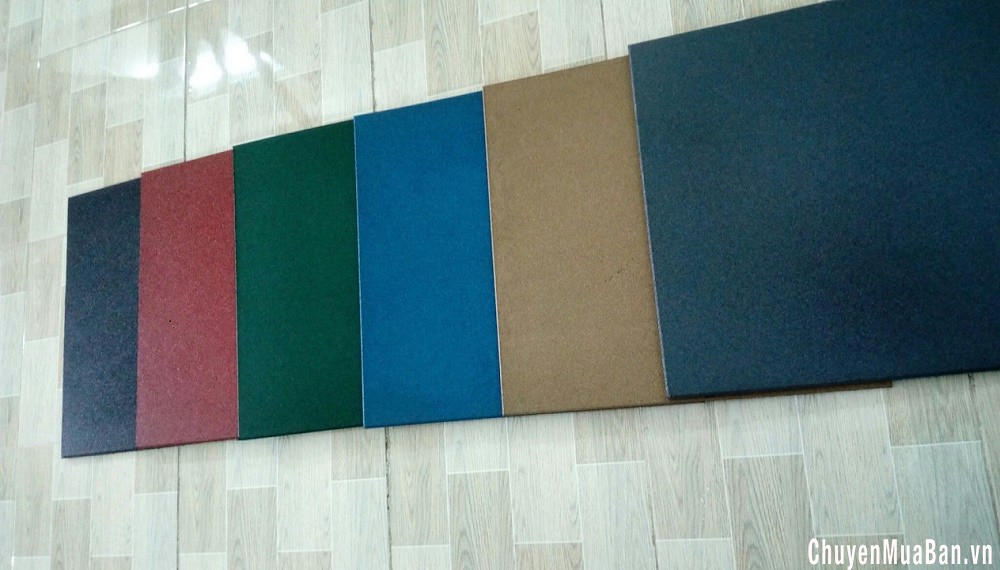This image captures a glossy, light brown tile floor with a noticeable light reflection and glare in the top left corner. On this floor, six colorful squares have been laid out in a staggered, overlapping sequence, extending from the upper right corner to the lower left center. The sequence begins with a nearly full dark blue square, followed by a partially obscured light tannish square underneath it. Next, a light blue square overlaps the previous one, followed by dark green, dark red, and finally a black square. The squares are described as colored pieces of board or tile. In the bottom left corner of the image, there is white text that reads "C-H-U-E-N M-U-A B-A-N dot V-N."